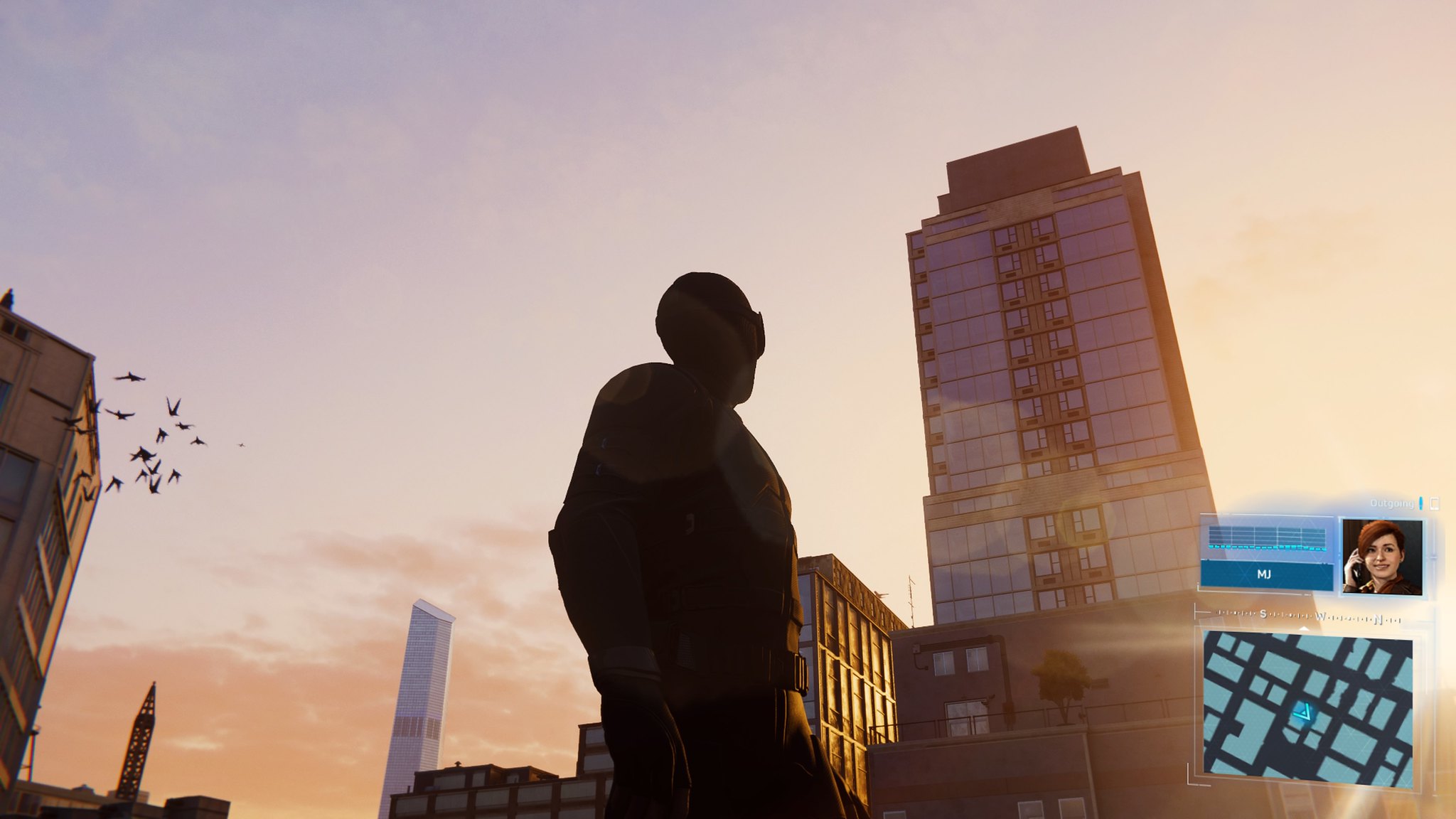A bustling urban cityscape fills the background, dominated by towering high-rises. On the right side, a prominent skyscraper with expansive glass windows catches the eye, while in front of it stands a shorter building that rises to about a quarter of the height of the larger structure. Nestled further in front is a smaller building, adding depth to the scene. Adjacent to these on the left, another high-rise adds to the dense skyline. 

In the center of the image, a silhouette of a person—with indistinguishable gender traits—stands prominently. The figure appears to be wearing long sleeves and possibly glasses. The left hand is visible, bathed in sunlight that streams through the surrounding structures, highlighting this area. The image is cropped at the person’s thighs, adding a sense of intrigue.

To the left, another building is visible, around which birds are flying, adding a touch of nature to the urban environment. A tower looms in the background on the left side, enhancing the cityscape's complexity. On the right side of the image, there's an insert with a light blue box that likely contains text and a picture. The text appears to say "Hi" in white, accompanied by an image of a woman with brown hair holding a telephone to her ear. Below this, another blue section with brownish stripes looks like it could be rafters of a building or another abstract pattern.

The sky above is a light blue, transitioning into a pinkish-yellow hue that suggests the sun has just set. The overall scene is enveloped in the subtle, warm glow of the dusk.